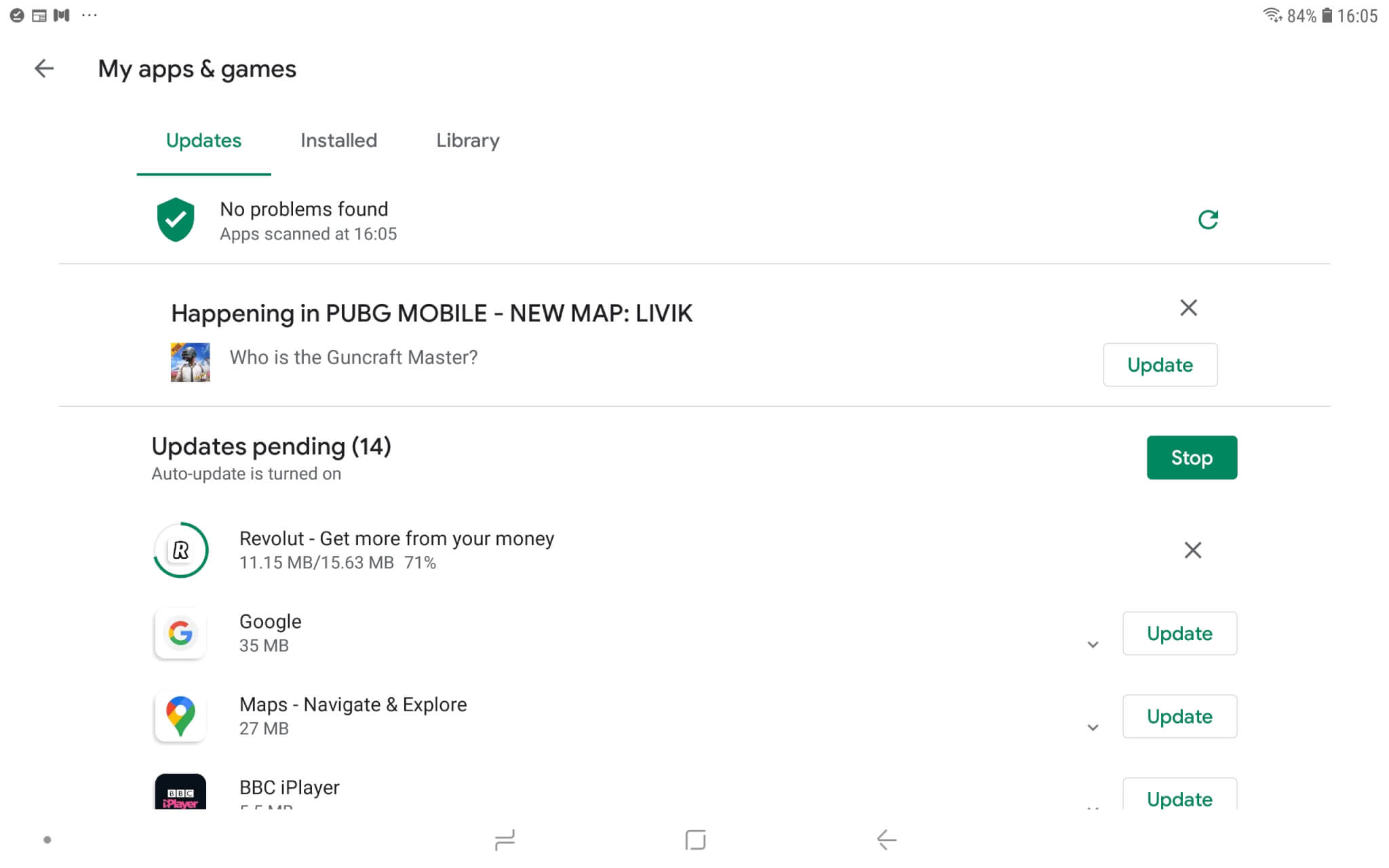This detailed caption describes a screenshot taken from an Android phone's "My Apps & Games" section, which is visible through a desktop interface. At the top left corner, there is a back button, and the title "My Apps & Games" is prominently displayed. Adjacent to it are three tabs: Updates, Installed, and Library, with Updates highlighted in green.

Below this, a status message reads, "No Problems Found, Apps Scanned at 16:05," alongside a green shield icon with a checkmark, indicating security. On the far right, there is a refresh button.

The next section features a notification for "Happening in PUBG Mobile" regarding a new map named LIVIK, with a dismiss option marked by a black X. This is followed by a query: "Who is the GunCraft Master?" and an update button on the right.

Further down, an update summary shows "Update Pending: 14" with a notification that "Auto-Update is turned on," accompanied by a green stop button. Directly beneath, the screen displays the Revolut app's promotion "Get more from your money," alongside a dismissable black X. The status of the app download for Revolut reads "11.15 MB/15.63 MB (71%)," indicating progress.

The following apps are lined up for updates, with each showing their respective sizes and update buttons. "Google" requires a 35 MB update, "Maps - Navigate & Explore" needs a 27 MB update, and the "BBC iPlayer" also has an available update button.